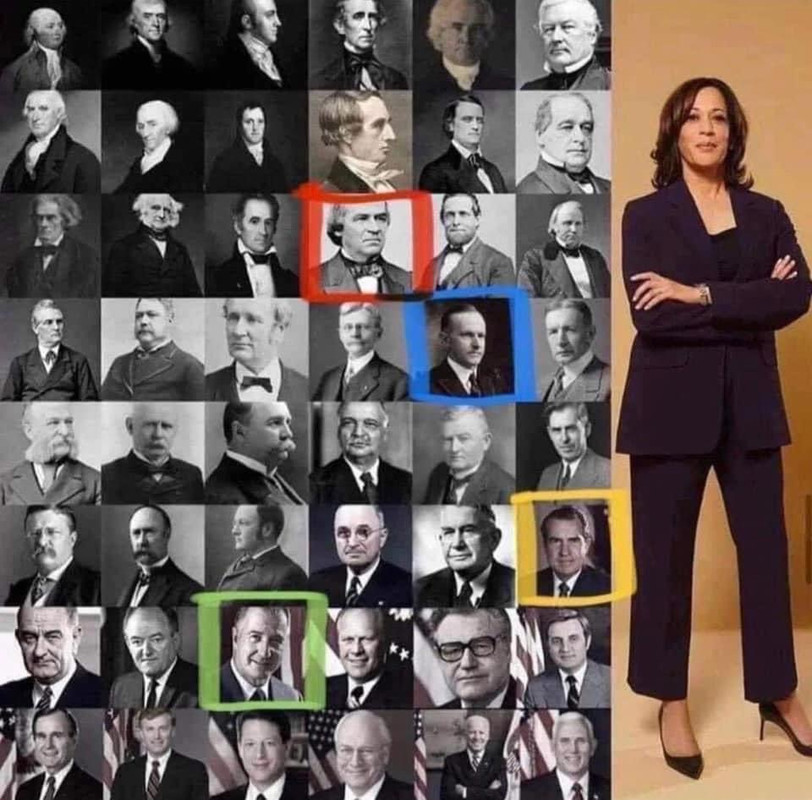The image on the left features a collection of numerous black-and-white photographs of U.S. Vice Presidents, arranged chronologically from the upper left, starting with the Vice President under George Washington, and continuing down to Mike Pence in the lower right. The first four images in the sequence are painted portraits, transitioning into actual photographs as time progresses. Several of these images are circled in various colors: Richard Nixon is highlighted with a yellow circle, Lyndon B. Johnson with a green circle, and two other unidentified vice presidents are marked with blue and red circles.

On the right side of the image stands a colored photograph of Vice President Kamala Harris. She is wearing a sleek black pantsuit paired with black high heels, exuding confidence with her arms crossed and a subtle, self-assured smile on her face. Her brown hair frames her tanned skin, adding to her composed and authoritative demeanor.